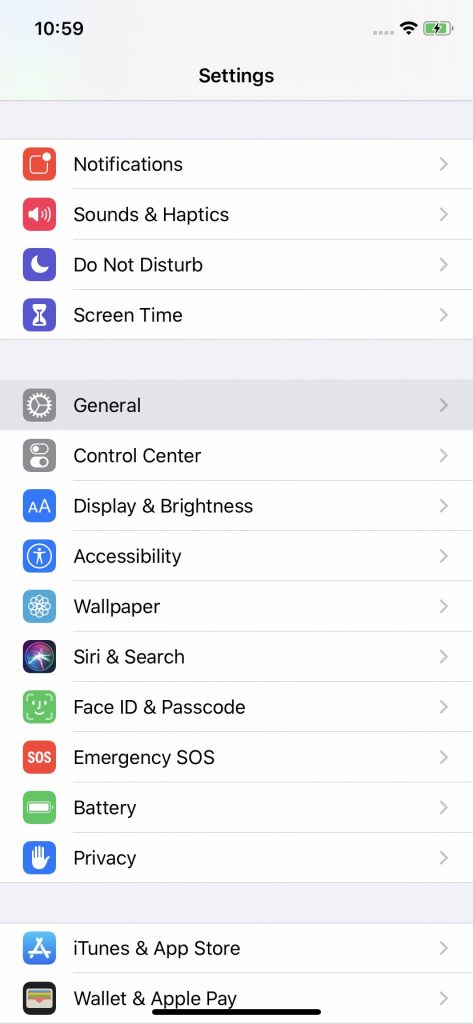The image is a screenshot of an iPhone's Settings menu. The screenshot prominently displays various options available under the device's settings, organized into a list format. The options visible in the list include:

- Notifications
- Sounds & Haptics
- Do Not Disturb
- Screen Time
- General
- Control Center
- Display & Brightness
- Accessibility
- Wallpaper
- Siri & Search
- Face ID & Passcode
- Emergency SOS
- Battery
- Privacy
- iTunes & App Store
- Wallet & Apple Pay

The settings interface is standard for iOS devices, presenting the user with a range of customizable features and controls to manage their iPhone's functionality, security, and user experience. The screenshot captures the meticulous organization and design of Apple's iOS Settings menu, highlighting the options available to the user for a personalized and secure phone setup.